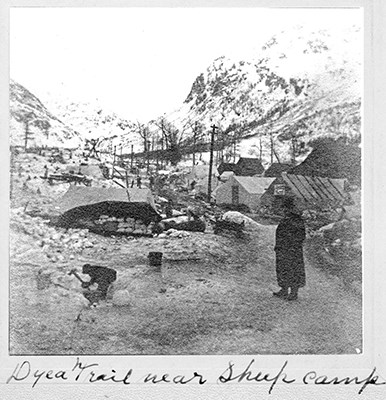This is a grainy, black and white photograph that appears to have been taken a long time ago, possibly with a Polaroid camera. The image is labeled in cursive at the bottom, which partially reads "DYEA Trail Near," although the text that follows is difficult to decipher. The scene depicts two figures standing on a road next to a makeshift campsite with tents and small buildings on the left. The first figure, located in the bottom right of the frame, is dressed in a long black coat and a top hat, looking away from the viewer. The second figure, slightly to the right, is the silhouette of a person holding a pickaxe, bent over as if mining. Further back, utility poles run through the scene towards a backdrop of towering, snow-covered mountains, which fade into a light white color against the sky. The entire photograph is slightly fuzzy and has a vintage, grainy texture that adds to its historical feel.